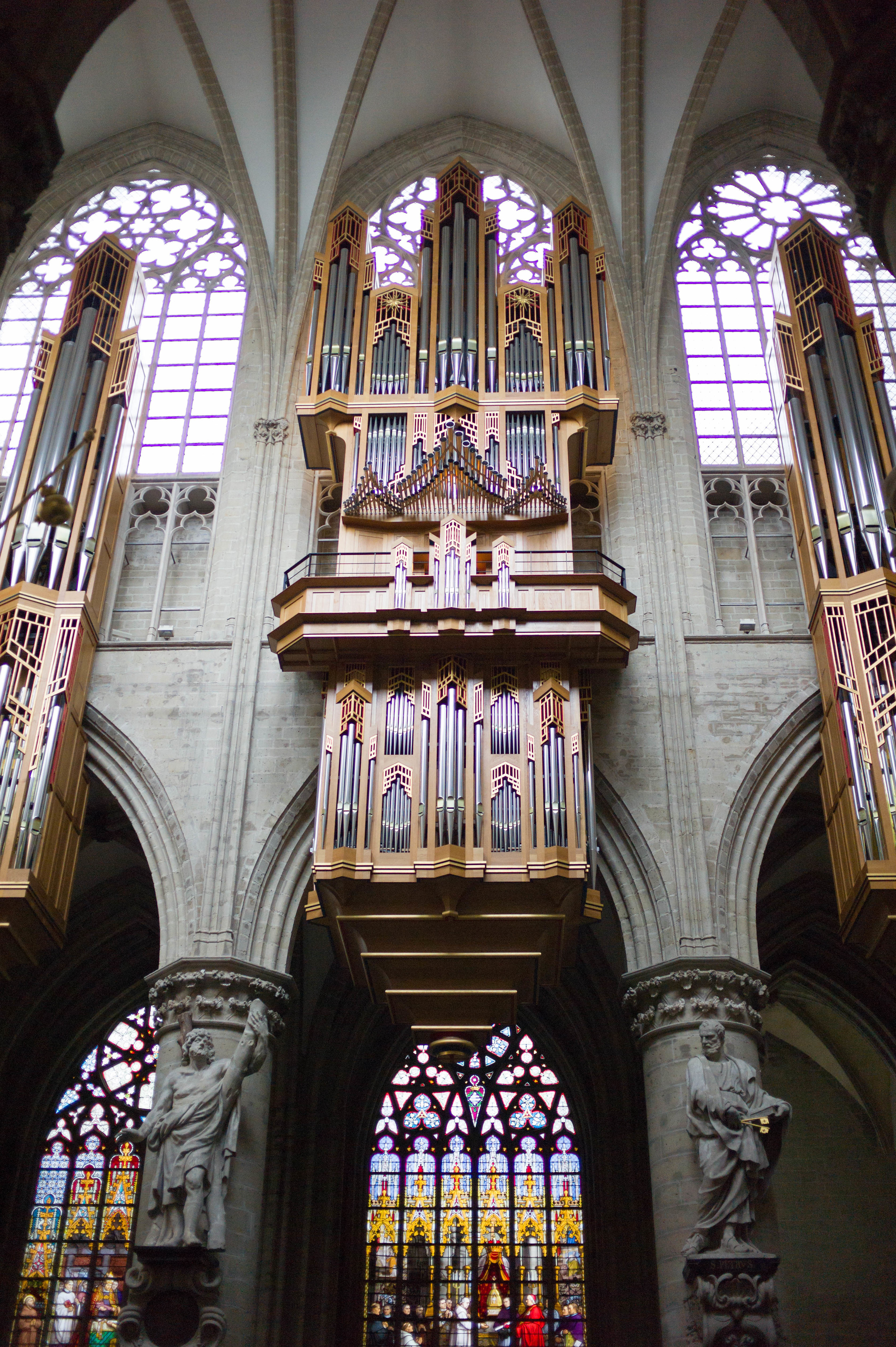This photo captures the grand interior of an ancient, well-preserved cathedral, estimated to be around 500 years old. Dominated by a massive, intricately carved organ with pipes arrayed in the center, left, and right, the scene exudes a sense of majestic antiquity. The cathedral's vaulted, white ceiling rises above a series of elegant archways, each flanked by statues holding various objects. Notably, one statue on the right seems to grasp a set of flags, adding a curious detail to the ornate surroundings. The lower section of the image reveals more statues adorning the middle left and right sections, while stained glass windows on the lower and left sides capture and scatter light, casting a multitude of colors upon the polished wooden surfaces. Golden decorative elements, resembling castle-like shapes, further embellish the walls, contributing to the cathedral's overall grandeur and timeless beauty.